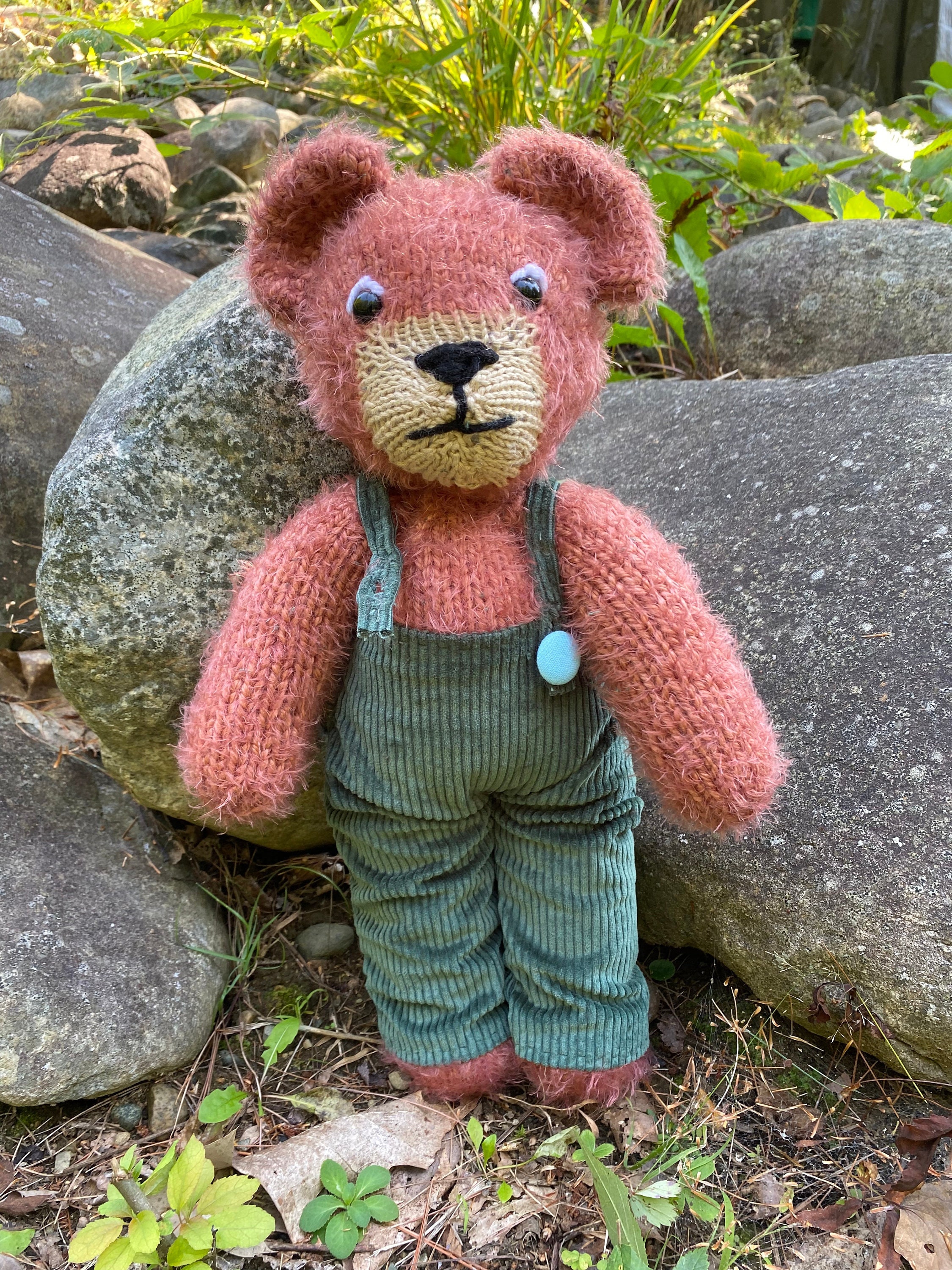In the photograph, a fluffy teddy bear with mauve-colored, crochet-like fur and soft, hair-like texture is prominently featured in an outdoor setting. This children's plush toy, which stands upright against a large rock, has distinct facial details: two black and white eyes, a beige-tan muzzle, and a crocheted black nose and mouth. The bear is dressed in bluish-green corduroy overalls with suspenders. In the background, several large rocks are visible amidst a lush environment filled with grass, weeds, bushes, and plant life. A tree trunk is also discernible. The sunlight gently illuminates the scene, indicating that the photo was taken outdoors during the daytime. The overall composition includes soil at the base and various stones scattered around, resembling a garden or forest area.